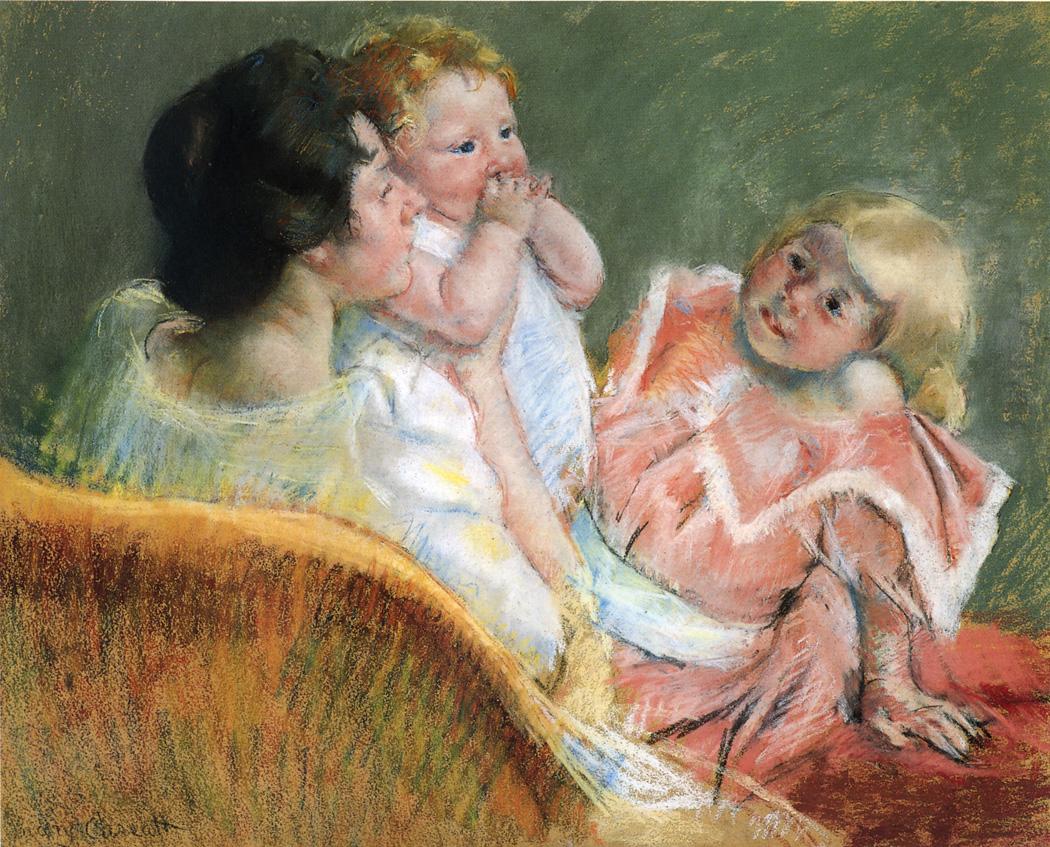This painting, likely from the medieval or early Renaissance era, depicts a serene domestic scene with a mother and her two children, which could be displayed in a museum featuring older works. The mother, positioned slightly to the right and partially turned away, has short, dark, pinned-up hair and is dressed in white. She tenderly holds an infant with curly blonde hair, also dressed in white. The infant has a chubby physique and blue eyes, exuding an innocent charm. Beside them, on the orangish-gold couch interspersed with green and darker red hues, sits a slightly older child, a young girl with longer brown hair. She is dressed in an orange and white outfit and is looking lovingly at her mother, her hand gently placed on her mother's knee. The background walls are a blend of green with hints of yellow or golden tones, contributing to the painting's warm, nostalgic ambiance.